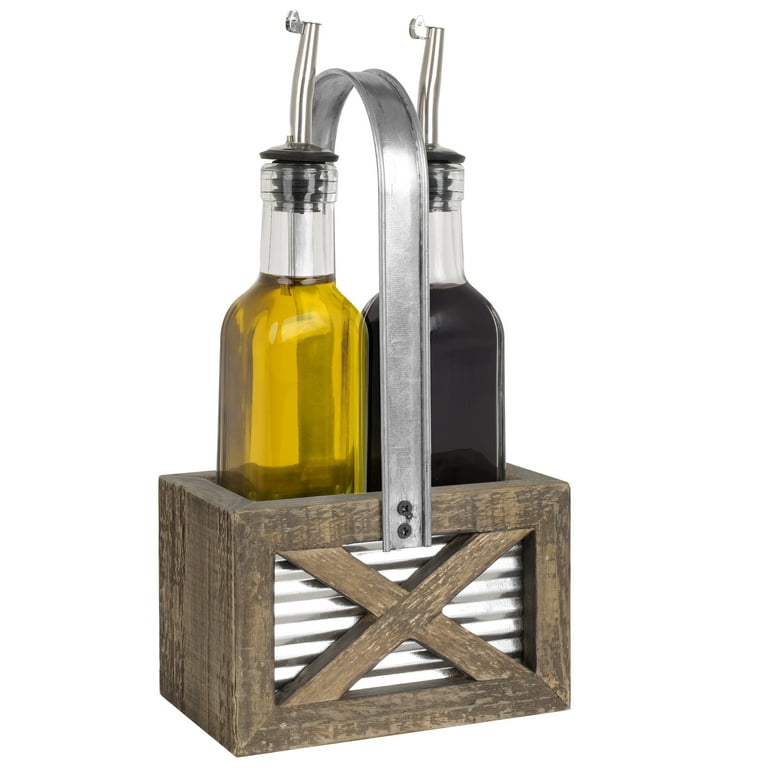The image showcases a detailed table setting item consisting of a pair of clear glass jars nestled within a wooden carrying tray. The tray extends halfway up the jars, with a wooden X design on its side and corrugated metal forming the background. A long, metal hoop handle arches between the two bottles, allowing for easy transport. The bottle on the left contains nearly full, yellowish olive oil, while the right houses dark brown-black balsamic vinegar. Each jar is fitted with a pour spout plug, enabling controlled dispensing of their contents.